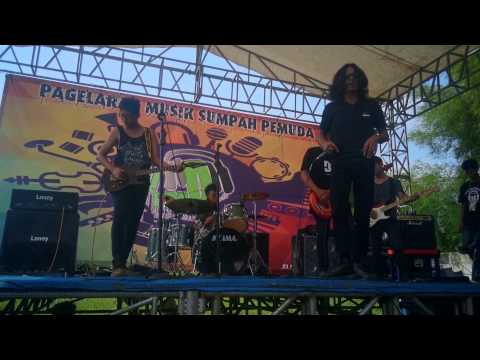The image captures a lively outdoor stage performance by a band under a yellowish beige tent. The scene is set against a backdrop of a clear blue sky and large green trees, indicating it's a sunny day. The stage features a diverse group of musicians: three men playing electric guitars—one with a black guitar, another with an orange guitar, and the third with a white guitar. There is also a long-haired male at the center with a tambourine standing at the microphone, adding vocals to the performance. In the background, a drummer is seated at a drum set, contributing to the rhythmic foundation of the music. To the right side of the stage, another individual appears to be joining the group. The backdrop features a banner with the words "Pagelar Musik Sumpah Pemuda" and displays images of various musical instruments, enhancing the musical ambiance of the scene. A blue mat is laid out on the stage, contrasting with the predominantly black stage floor.